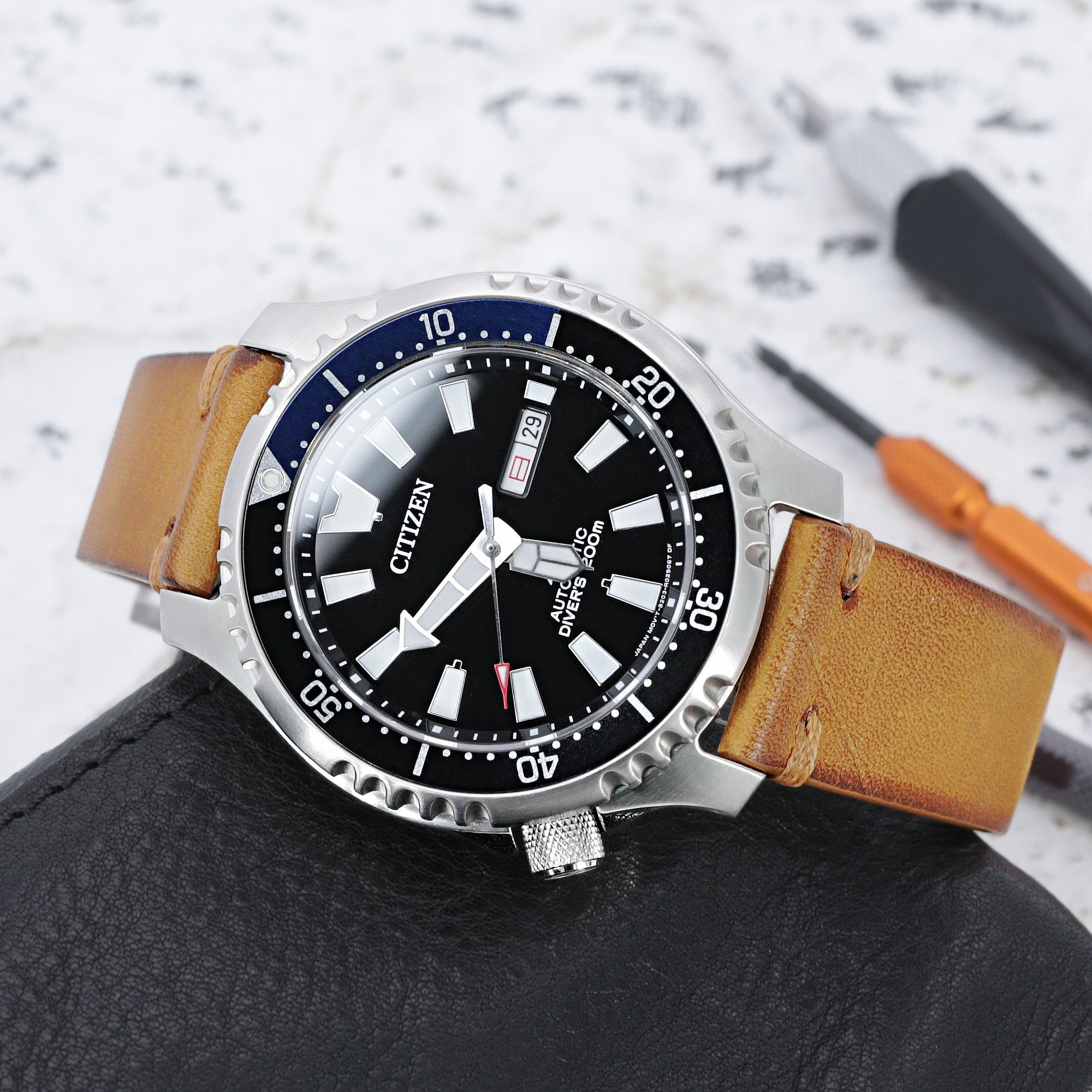This high-quality stock image features a Citizen men’s analog watch prominently in focus, positioned on a black leather surface, possibly a wallet. The watch, with a large, black face and silver dial, showcases thick, wide, luminescent silver hands with a slender second hand that has a red tip. The date display reads '29,' and the watch includes text that says "Diver’s 200 meters," indicating its water resistance. Surrounding the black face is a rotating silver bezel. The band is brown leather, adding to its sophisticated design. The blurred background includes a white, granite-speckled countertop, along with an orange-handled tool and a black-handled tool, suggesting a watch repair setting.